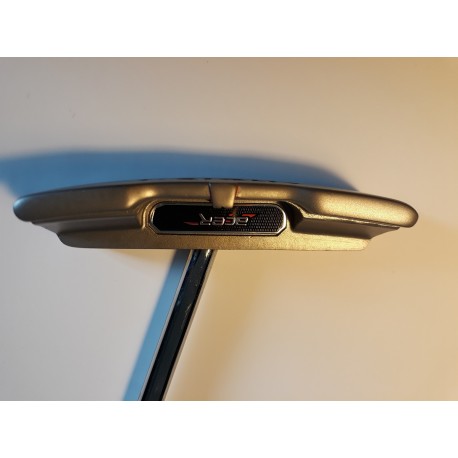The image depicts a cylindrical, upside-down gray electrical device, possibly an electronic appliance like a modem, vacuum cleaner, or router, situated against an off-white wall. The device, made of metal, prominently displays the brand name "Acer" in silver letters on a horizontal black section, although the branding appears upside down. Extending from the device is a silver metal rod angled up and to the right, contributing to the overall industrial look. The surrounding setting is minimal, casting a shadow on the wall behind, further emphasizing the metallic and sleek design of the equipment. The device's construction includes a middle grill and a handle, enhancing its intricate details and build.